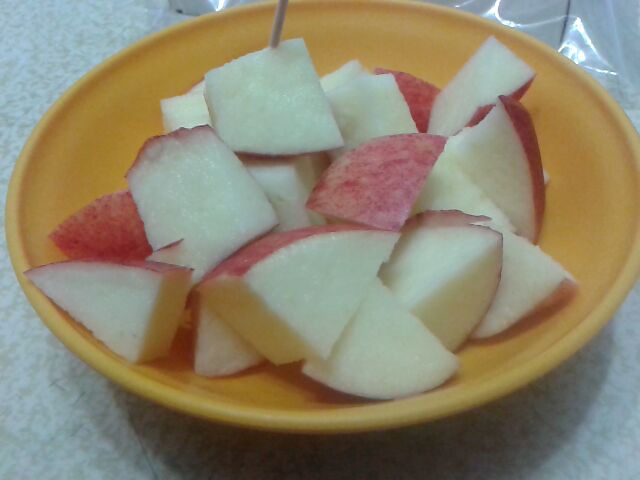This image features a medium-sized, orangish-yellow ceramic bowl filled with freshly cut apple chunks. The apples, likely Gala or Red Delicious, exhibit a crisp white interior and vibrant red and yellow-tinged skin, suggesting they are very fresh and juicy. Each piece is bite-sized, approximately one-inch squared, maintaining their natural rounded edges. A solitary toothpick pokes out from one of the apple chunks, hinting at the possibility of the apples being presented as hors d'oeuvres. The bowl rests on a grayish, marble-like countertop or surface, which has a slightly murky appearance. In the background to the right, a piece of clear plastic wrap or a Ziploc bag is visible, possibly indicating the apples were recently stored in it.